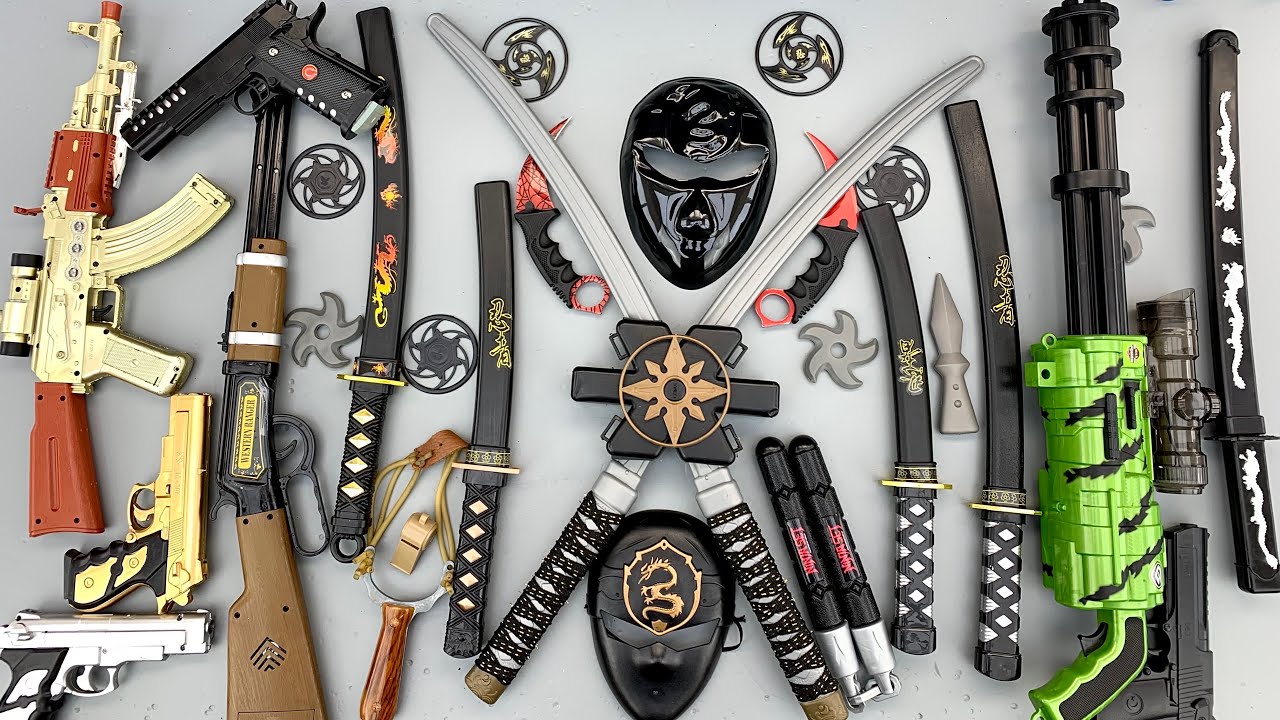This captivating photograph showcases a meticulously organized collection of assorted plastic weapons arranged against a solid white gradient background. Central to the composition are two intricately designed katanas, crossed in the middle and flanked by a pair of black ninja masks adorned with unique dragon emblems. Surrounding these focal points are a variety of weaponry, including multiple rifles—the hunting rifle on the left distinguished by an orange tip, indicating its fake nature. A formidable green and black minigun with a detailed handle and barrel stands on the right, complemented by an array of handguns in gold and standard black, with one particular pistol prominently featuring a sniper scope. The collection also boasts traditional ninja tools such as nunchucks, black and gold pin-striped shurikens, sais, and two red and black karambits. Additional items include a slingshot and several sheathed samurai swords, exhibiting black covers decorated with intricate yellow, red, and white designs. The assortment is thoughtfully spaced, ensuring each weapon—whether gun, sword, or throwing star—is distinctly visible and easily identifiable.